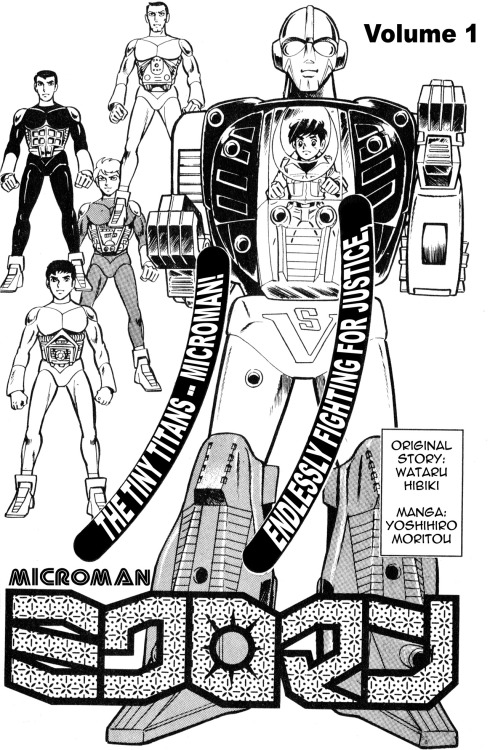The image is a black-and-white cartoon cover, likely for a comic book or manga titled "Microman." At the top right, "Volume 1" is prominently displayed. On the left side of the cover, there are four men arranged vertically: the top and bottom figures are dressed in white, while the second man from the top is in black and the one below him is in dark gray. To the right of these men stands a larger robot, with a man visible inside a chest window, appearing to control the robot. The title "Microman" is featured prominently, with an additional phrase "The Tiny Titan's Microman" in white letters on black banners. Beneath the title, probably in Japanese or another Asian language, are more texts. Another banner reads, “Endlessly Fighting For Justice.” In the bottom right of the cover, a text box credits the original story to Wataru Hibiki and the manga work to Hoshihiro Morito. The entire image is detailed yet monochromatic, adding to its dramatic flair.